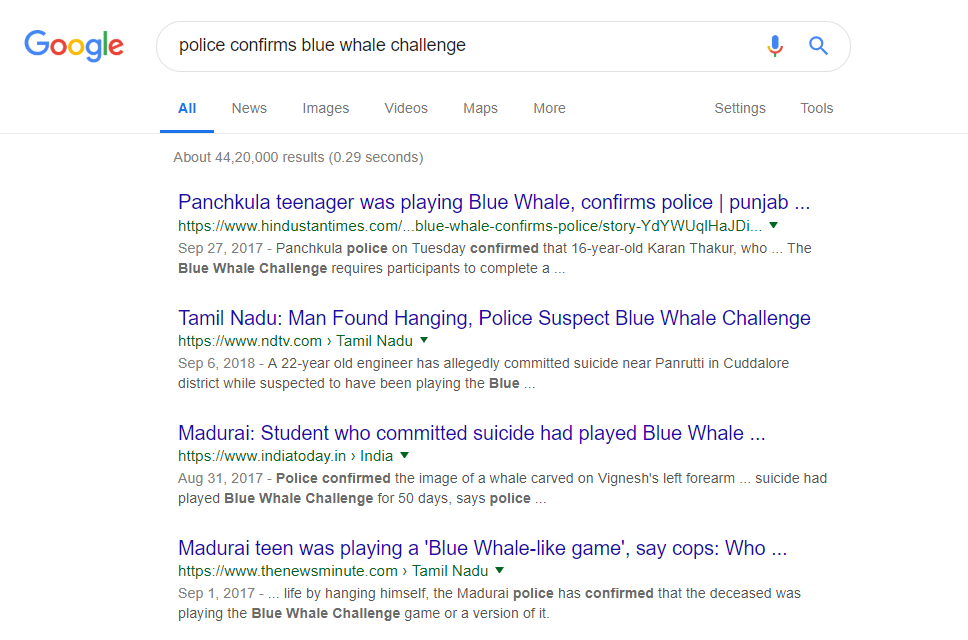In this image, you are looking at the results displayed in the Google search bar. The search term "Police Confirms Blue Whale Challenge" is typed in and highlighted in blue. The search results feature four prominent entries, all related to the Blue Whale Challenge and its implications, dated from 2017. 

1. The first result reads: "Panchkula teenager was playing Blue Whale, confirms police."
2. The second result states: "Tamil Nadu man found hanging; police suspect Blue Whale Challenge."
3. The third entry highlights: "Madurai student who committed suicide had played Blue Whale."
4. The fourth result mentions: "Madurai teen was playing a Blue Whale-like game, say cops."

Each entry suggests tragic incidents linked to the Blue Whale Challenge, underscoring the pervasive concerns around the online phenomenon during that year.